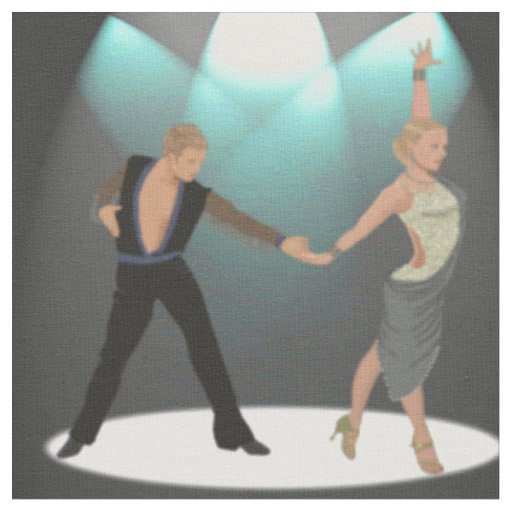The image is an illustrated scene featuring a male and female dancer performing under an array of bright, colorful lights, evoking a theatrical ambiance. Both dancers have white skin and blonde hair. The man is dressed in black attire, including black trousers and shoes, with a vest that has brown sleeves. He is extending his left hand outwards to hold the woman's right hand, while she has her left hand raised towards the ceiling. The woman is adorned in a shimmering silver top paired with a grey skirt, and she is wearing brown shoes. They are positioned within a vividly lit, circular stream of light, suggesting a stage setting. Above them, three distinct rays of light—blue and white—illuminate the scene, contributing to the contrast against the dark background. Despite the vibrant setting, the image retains a slightly blurry quality, enhancing its artistic, possibly computer-generated or cartoon-like, style. The dancers' dynamic poses and intense focus on their interaction imply a moment of graceful choreography, with the man looking down at their intertwined hands as the woman twirls, her back partially facing him.